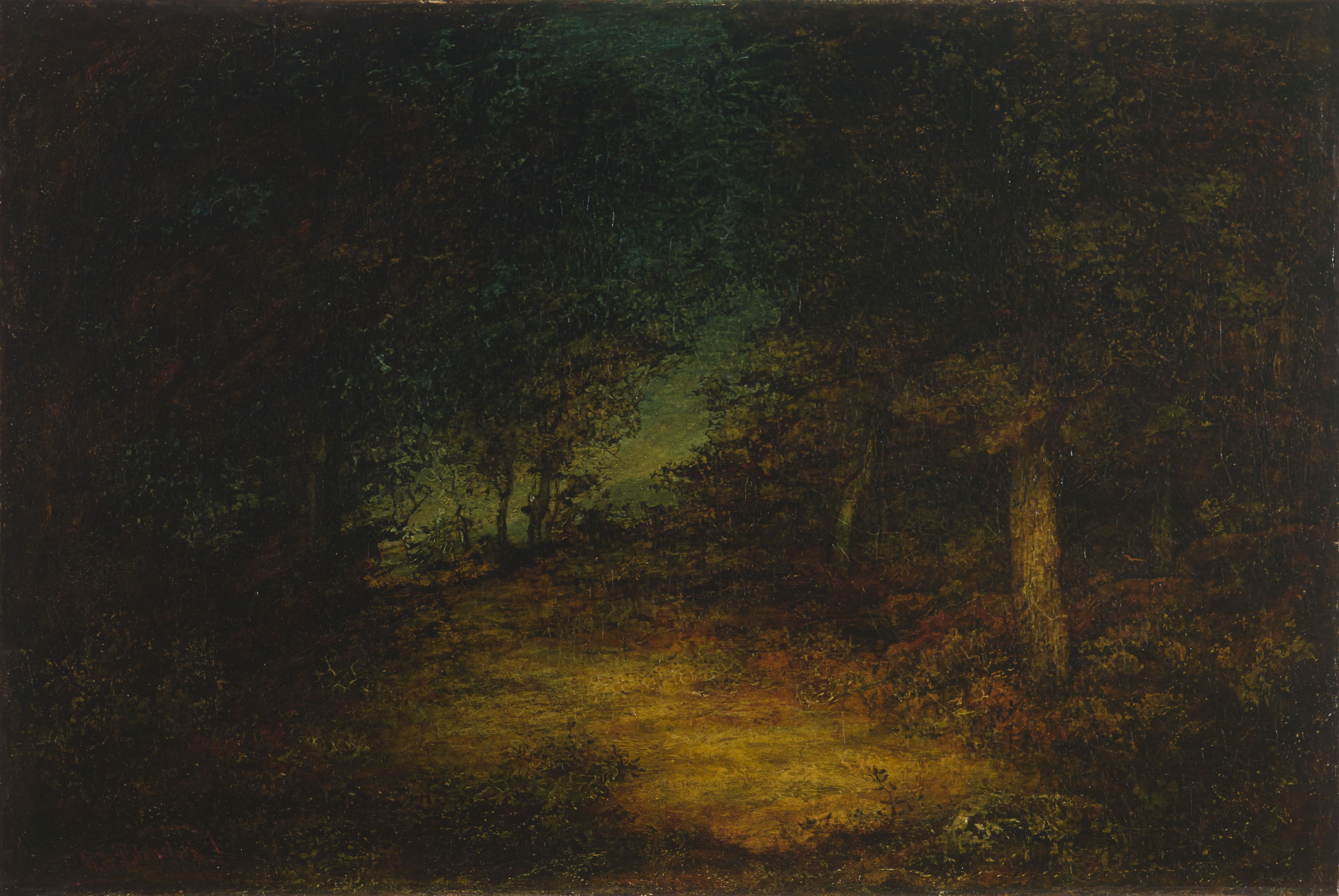This horizontally aligned, dark painting presents a somber, somewhat spooky yet sacred depiction of a forest at dusk or nighttime. The forest scene is dominated by tall trees with abundant branches and leaves, creating a dense canopy that obscures much of the light. The colors primarily used are various shades of green, blue, and golden yellow, with the sky exhibiting a gradient from a dark greenish-blue at the top to a lighter, greenish-yellow hue near the horizon.

In the center of the artwork, a light golden-brown dirt pathway cuts through the forest, leading to a small, illuminated meadow or glade. This area stands out with its golden-yellow and yellowish-green tones, contrasting with the darker surroundings. The forest floor is covered with leaves in hues of orange, brown, and black, enhancing the painting's dark, mysterious atmosphere.

There are no figures, animals, or man-made structures within the scene, emphasizing the isolation and quietness of this forested area. The meticulously detailed tree trunks and underbrush are revealed in shades of dark brown and black, with some lighter highlights that mimic the pathway's illumination. Overall, the painting is a captivating portrayal of nature's beauty and serenity under the cloak of night.